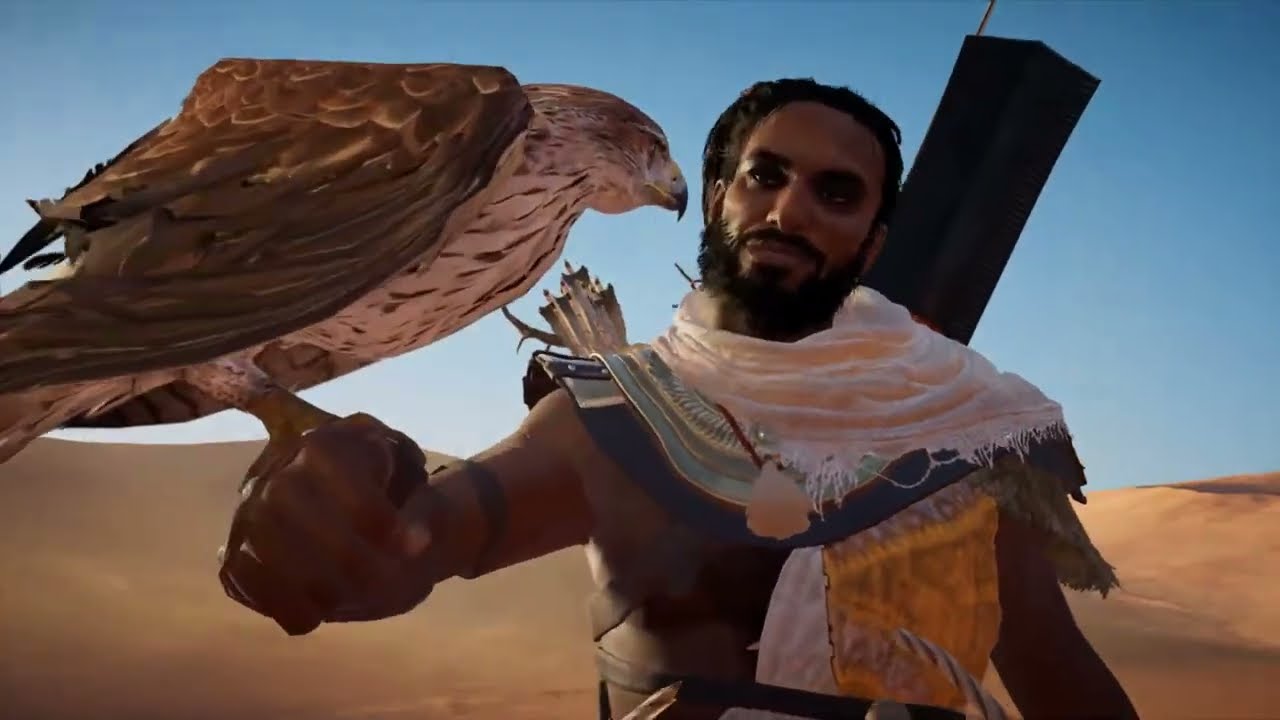This image appears to be a screenshot from a video game, showcasing a character who is a Middle Eastern man with dark skin, black hair slicked back, and a prominent black beard. He is standing in a desert environment, with rolling sand dunes beneath a bright blue sky. The man is dressed in a striking ensemble: a white scarf is draped elegantly around his neck, overlaying a thick, detailed armor that features shades of brown, yellow, and hints of metallic blue and silver. A leather strap circles his waist, and a quiver of arrows with visible feathers is positioned over his right shoulder, hinting at the presence of a bow behind him.

The character is facing slightly to the right, about the three o'clock position, with just his torso visible. His right arm is extended outward, donning a glove. Perched majestically on this glove is a falcon with its eyes closed. This bird features a yellow tail, white breast speckled with brown, dark brown wings, and a yellow beak tipped with black. The falcon's wings are folded neatly against its body. The overall composition evokes a sense of pride and readiness, with the character gazing intently at the falcon as if sharing a deep, unspoken bond.